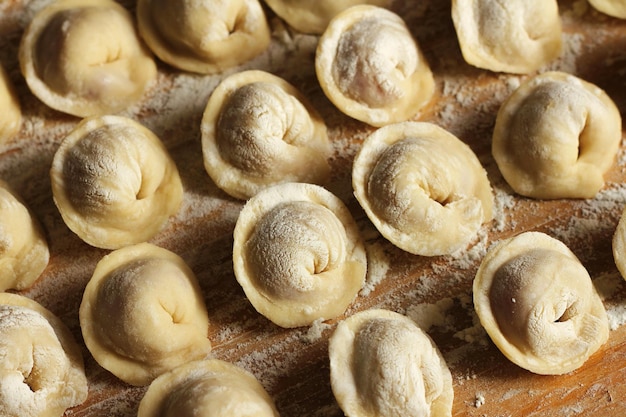The photograph features a batch of small, circular food items, likely homemade ravioli or a similar dough-based dish, arranged neatly in rows on a light brown wooden surface that resembles a cutting board. There are approximately 15 to 16 of these dough pieces, organized in 3 to 4 rows that run diagonally from the lower left to the upper right of the image. Each piece is light brown or cream in color and has a distinctive ring with a small belly-button-like indentation at the center, indicating they are unbaked and filled. The surface and the dough items are dusted with a generous sprinkling of white flour, giving the scene an artistic, rustic feel.